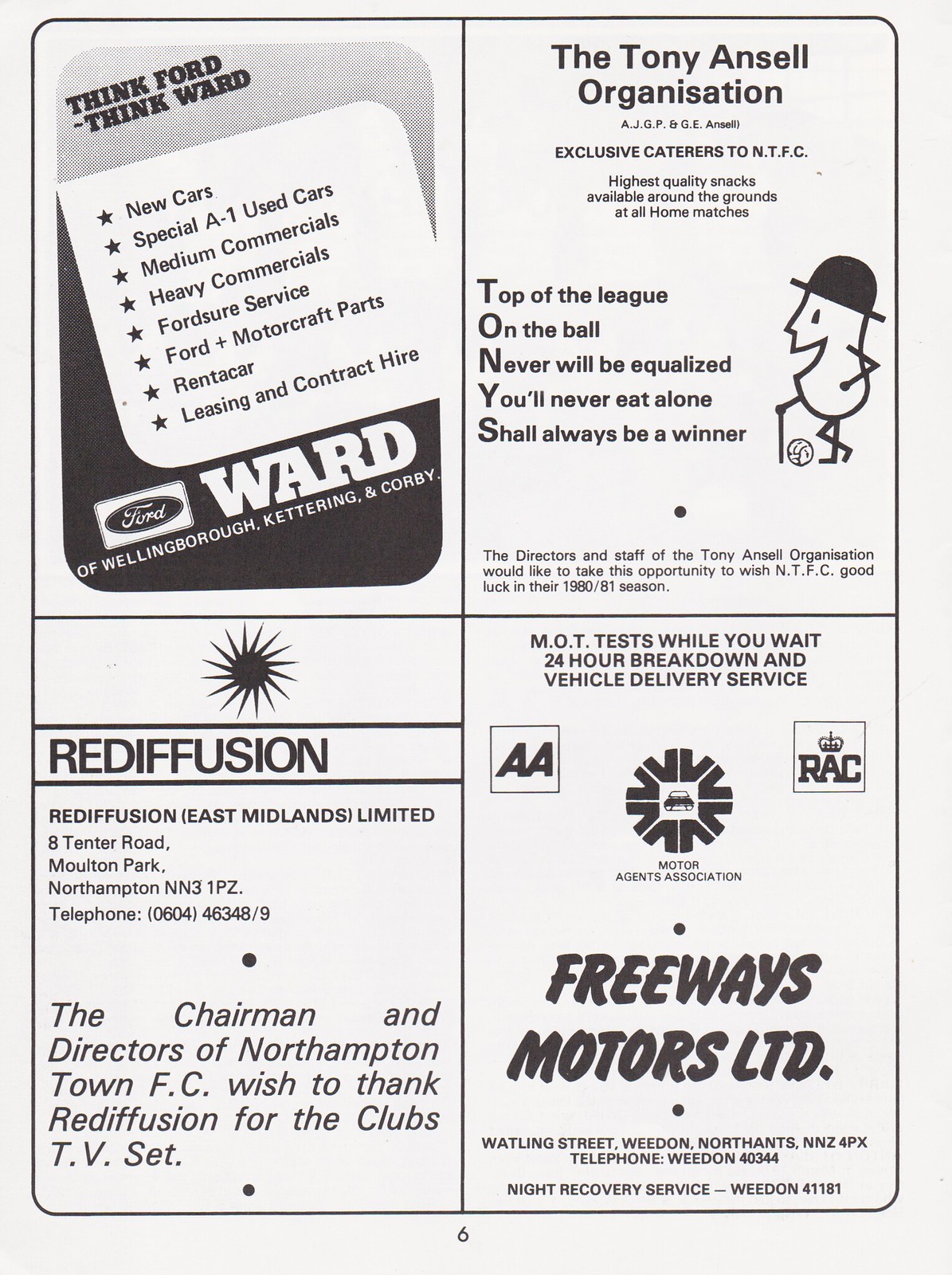The image is a black-and-white page that appears to be from an old magazine or newspaper, showcasing four different advertisements. The layout is divided into four roughly equal sections, two on top and two on the bottom. 

The top left section is an ad for the Ford auto dealer Ward of Wellingborough, Kettering, and Kirby, prominently featuring the slogan "Think Ford, Think Ward." The advertisement lists various services including special A1 used cars, medium and heavy commercials, leasing and contract hire, and mentions Ford service and Motorcraft parts.

The top right section highlights the Tony Ansell Organization, accompanied by a cartoon character reminiscent of Mr. Peanut wearing a hat. The text reads: "Top of the league, on the ball, never will be equalized, you'll never eat alone, shall always be a winner."

In the bottom left section, there is an advertisement for Rediffusion East Midlands Limited, providing their address as 8 Tenor Road, Moulton Park, Northampton, NN13 1PZ. The ad includes a note of gratitude from the chairman and directors of Northampton Town FC, thanking Rediffusion for the club's TV set.

The bottom right section features an ad for Freeways Motors Limited, which includes services like MOT test while you wait, 24-hour breakdown, and vehicle delivery service. The company's icon, address, and phone number are also present. Additionally, the page number "6" is visible at the bottom.